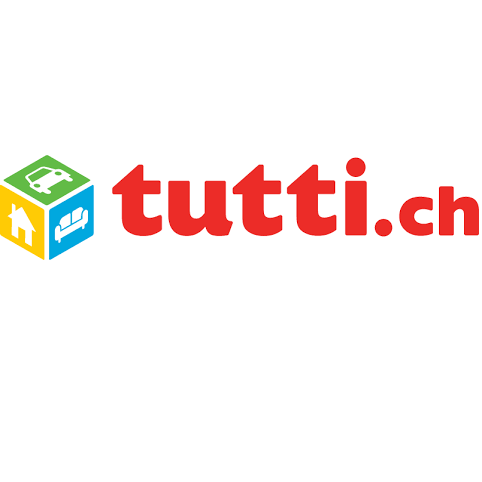This digital image features a simple, yet detailed company logo with no background, just a clean white canvas. The logo is horizontally aligned with a colorful cube-shaped icon on the left and bold red text on the right. The cube displays three distinctly colored sides: a green top with a white car silhouette, a yellow left side with a white house silhouette, and a blue right side with a white couch silhouette. Adjacent to the cube, in large, bold red letters, is the text "TUTTI.CH," likely referencing the company's website. The overall design is straightforward, focusing attention on the vibrant icon and the clearly legible URL.